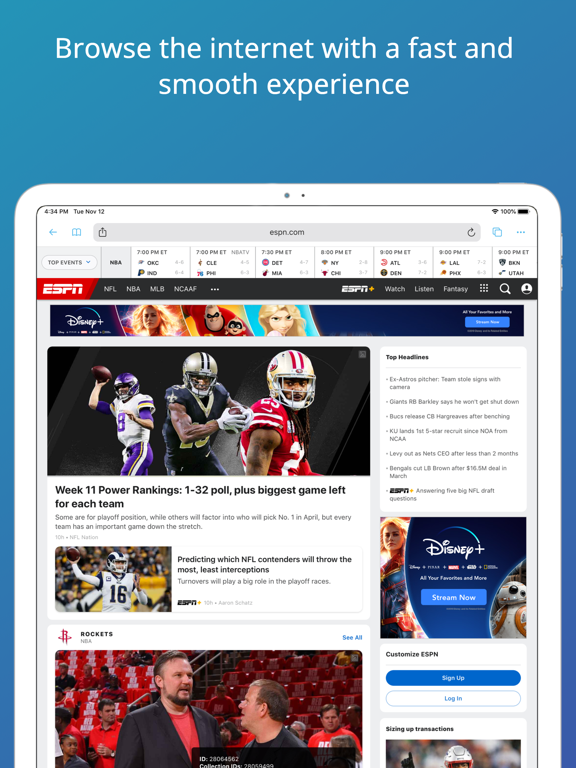**Caption:**

A detailed view of an ESPN interface on a white iPad, captured at 4:34 PM on November 12th, with a battery life of 100%. The interface showcases the homepage of espn.com, featuring a search bar at the top. Below the search bar, "Top Events" is highlighted on the left with live updates on NBA scores. Teams like the Oklahoma City Thunder against the Indiana Pacers are displayed with their current standings and game times.

Further down, there is the iconic ESPN logo bordered in white and red, accompanied by category tabs for NFL, NBA, MLB, NCAA Football, ESPN+, Watch, Listen, Fantasy, and a login option. An advertisement for Disney+ is prominently placed below these tabs, highlighting the bundle offer with Hulu and ESPN.

Continuing the sports updates, the interface displays NFL Power Rankings for Week 11, listing all 32 teams based on their current standings. Adjacent to this section is a feature on NFL contenders and information about the Houston Rockets NBA team's latest news.

To the right, the "Top Headlines" section lists five leading stories of the day. At the bottom right, there is another Disney+ advertisement promoting streaming options, positioned above sign-up and login links.